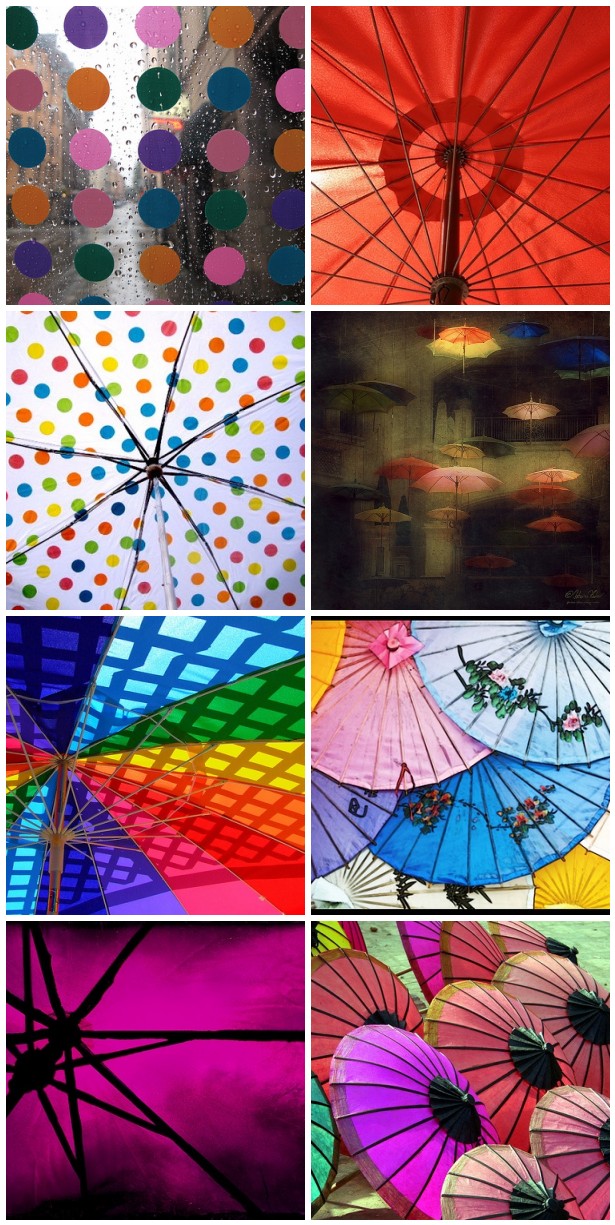This is a collage composed of eight smaller square photographs, each featuring various vibrant umbrellas and parasols. The arrangement consists of two columns with four rows. 

In the top-left image, a clear umbrella with multicolored polka dots in shades including purple, orange, pink, deeper pink, and green is featured against a rainy cityscape background, giving the perspective of looking through the umbrella. Adjacent to it on the right, the second image displays the underside of a red umbrella, revealing silver supports and a black handle with a dark maroon circle at the center.

The third image, positioned below the first, shows the inside of a white umbrella adorned with multicolored polka dots—each dot in hues of red, blue, green, orange, yellow, and various shades of blue—with black rods and a white pole. To the right of this, the fourth image is an artistic depiction of umbrellas floating through the air against an olive-green background. The umbrellas here are painted in diverse colors including pink, blue, navy blue, orange, yellow, green, dark green, red, and hot pink.

Continuing downward, the fifth image on the left presents a real umbrella seen from underneath, showcasing a rainbow array of colors arranged in a grid-like pattern and supported by bronze mechanisms. Moving right, the sixth image captures a collection of romanticized, pastel-hued Japanese-style parasols viewed from above, with prominent floral designs on some of them. The colors range from orange, pink, and light blue to navy blue, purple, and yellow with intricate details.

In the bottom-left corner, the seventh image captures the underside of a dark magenta umbrella in shadow, highlighting black support structures. The final, eighth image on the bottom right illustrates a side view of multiple stiff, unfurled parasols resembling paper umbrellas. They are predominantly pink and purple, some with bronze outlines and accents, displayed next to each other in a pleasing array.

This detailed collage captures an eclectic mix of umbrellas in various artistic and photographic styles, celebrating their colorful and functional diversity.